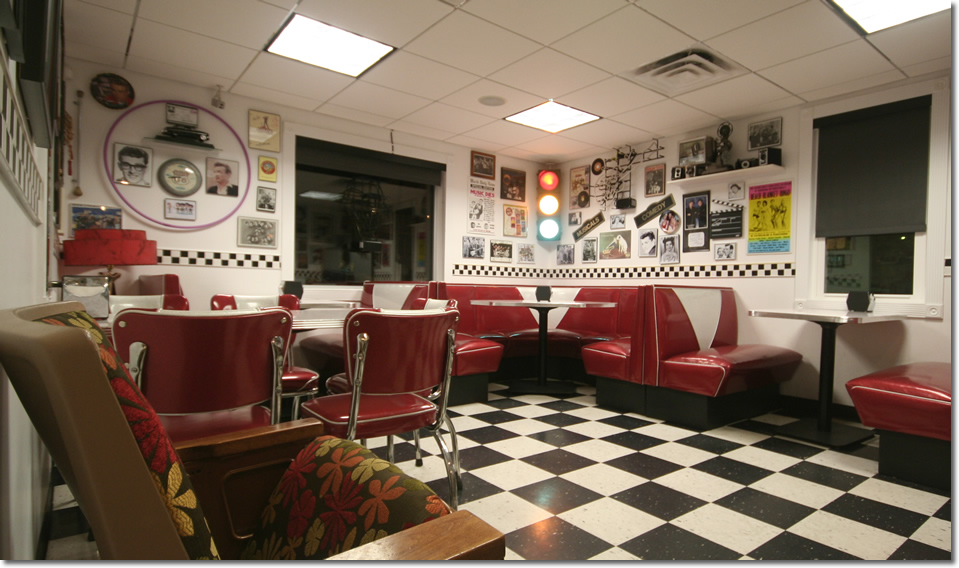The photograph captures a nostalgic, old-fashioned diner reminiscent of the 1950s. The interior features distinct elements that evoke the charm of that era. The ceiling is a white drop-down style with strategically placed squares allowing LED lighting to shine through. The walls are uniformly painted white, adorned with a black and white checkerboard trim running horizontally through the center. They are covered with an eclectic mix of vintage posters, images, and photographs, including iconic figures like Buddy Holly and Elvis Presley, enhancing the retro vibe.

In the far corner, a unique traffic light with all three signals—red, yellow, and green—illuminated adds to the quirky ambiance. The floor mirrors the wall trim with a classic black and white checkered tile pattern. Seating arrangements include multiple benches and chairs along the walls, all upholstered in red vinyl with white trim, echoing the style of the era. The diner features cedar booths for two along the far left and right walls, a round booth with a matching table in the corner, and red chairs with single-leg tables topped with white surfaces. This meticulously styled decor encapsulates the essence of mid-20th-century American diners.